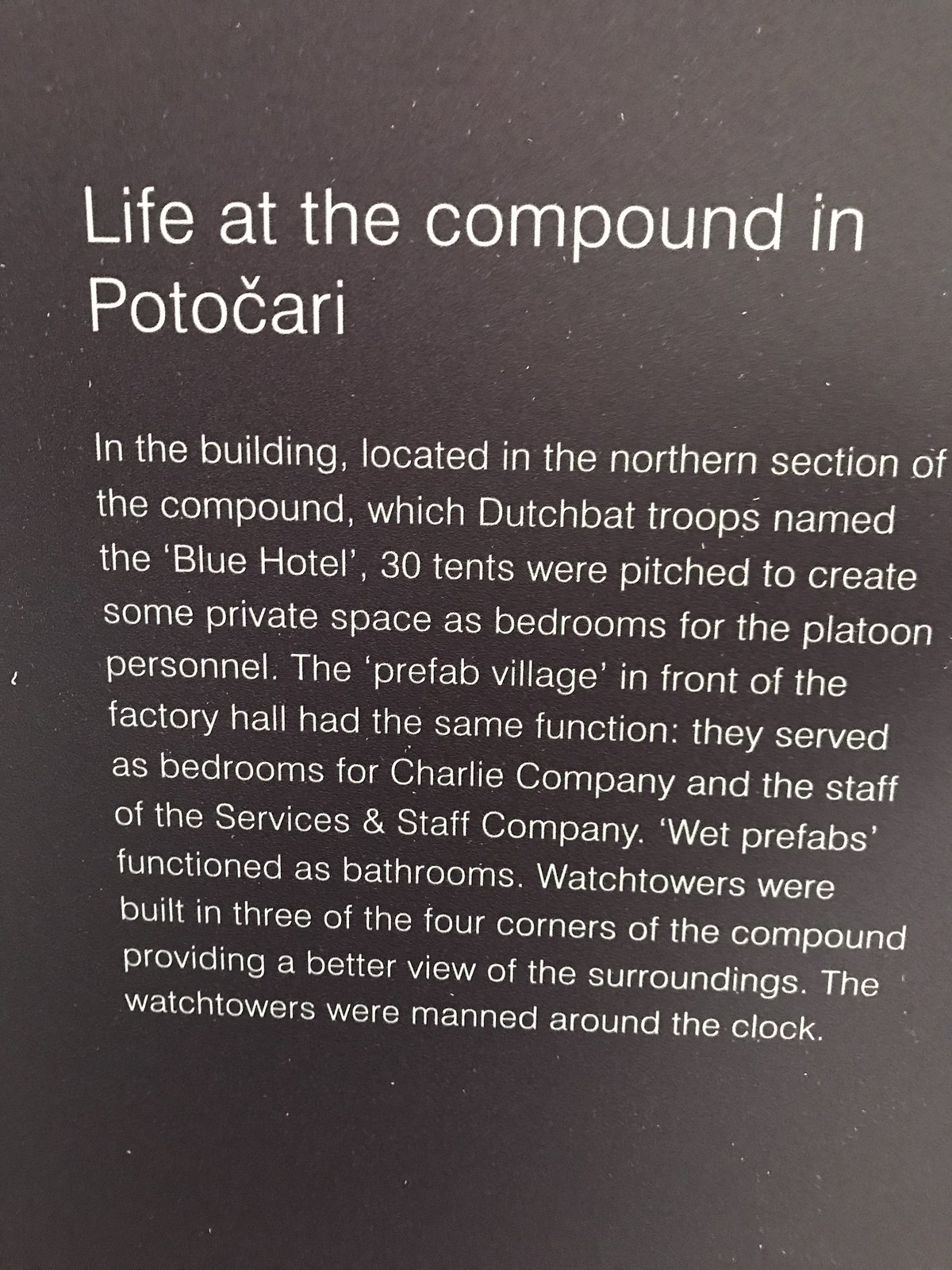The image depicts a horizontally rectangular, almost square, plaque or sign with a simple, dark gray background and white text. At the top in large letters, it reads "Life at the compound in Potocari." Below, in smaller text, it details the daily life at the compound: "In the building located in the northern section of the compound, which Dutch bat troops named the Blue Hotel, 30 tents were pitched to create some private space as bedrooms for the platoon personnel. The prefab village in front of the factory hall served the same function, providing bedrooms for Charlie Company and the Services and Staff Company. Wet prefabs functioned as bathrooms. Watchtowers were built in three of the four corners of the compound, providing a better view of the surroundings and were manned around the clock." The sign has no borders on any side and occupies the entire frame of the picture.